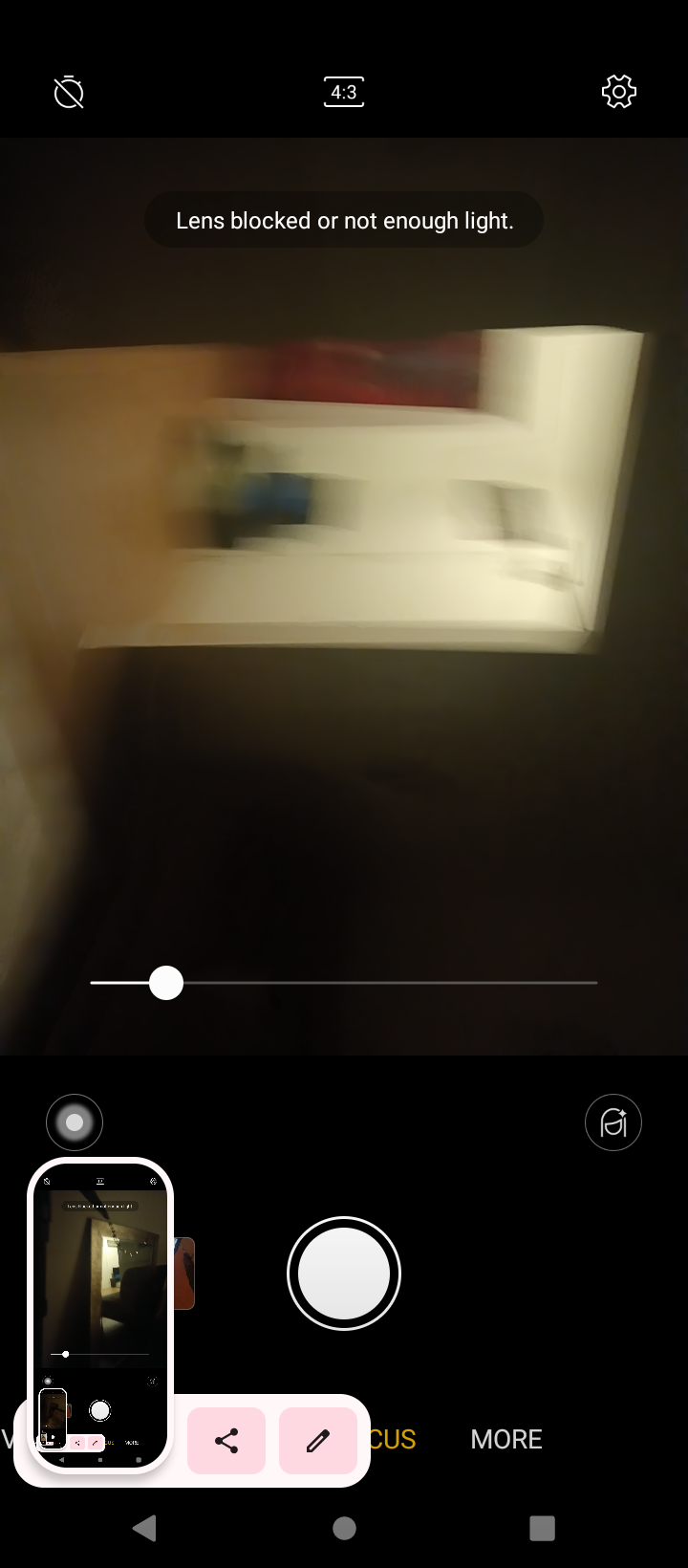The image depicts a smartphone screen focused on the camera application. The camera is attempting to capture a picture of a document placed on a table, but the image is significantly blurred. A warning message prominently displayed at the top reads, "Lens blocked or not enough light." The interface also provides quick access to settings. Interestingly, the screen showcases a "picture-in-picture" effect, where there is an inset image displaying a phone, which is itself capturing the same scene, creating a recursive visual of the phone showing an image of another phone, repeated endlessly. This visual effect adds a unique and intriguing layer to the otherwise simple scene of a camera's struggle to focus.